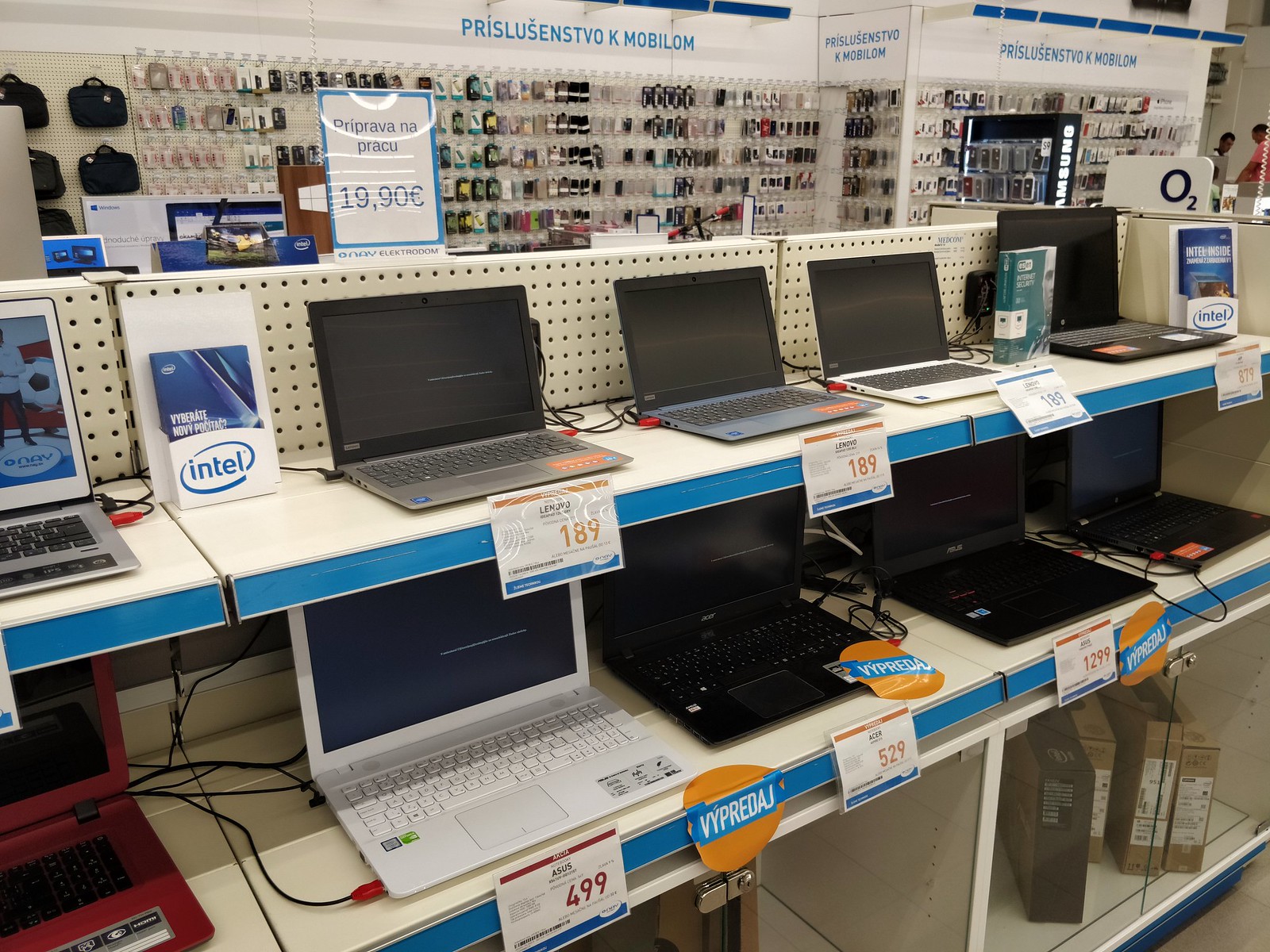This photo captures the interior of a tech store, likely a computer or electronics store located in a Slavic region but using Euro currency, as indicated by the prices on display. Prominently featured are two shelves stocked with a variety of laptops and Chromebooks, all opened and powered on except for one in the far left corner, which displays an "One" with a soccer ball icon on its screen. The laptops come in different colors, including black, white, and even a red one. Prices for these laptops range from €189 to €1,299. Each laptop has a small, detailed description tag and price in front of it, though the text is too small to decipher clearly. To the left, a sign with the Intel logo is visible, while a sign marked O2 is on the right. In the background, assorted mobile phones, computer accessories, and possibly laptop bags with handles can be seen on the shelves. Underneath the display shelves are some empty boxes, possibly meant for laptops. The store is illuminated with various electronic gadgets visible, creating a detailed snapshot of a typical electronics retail environment.